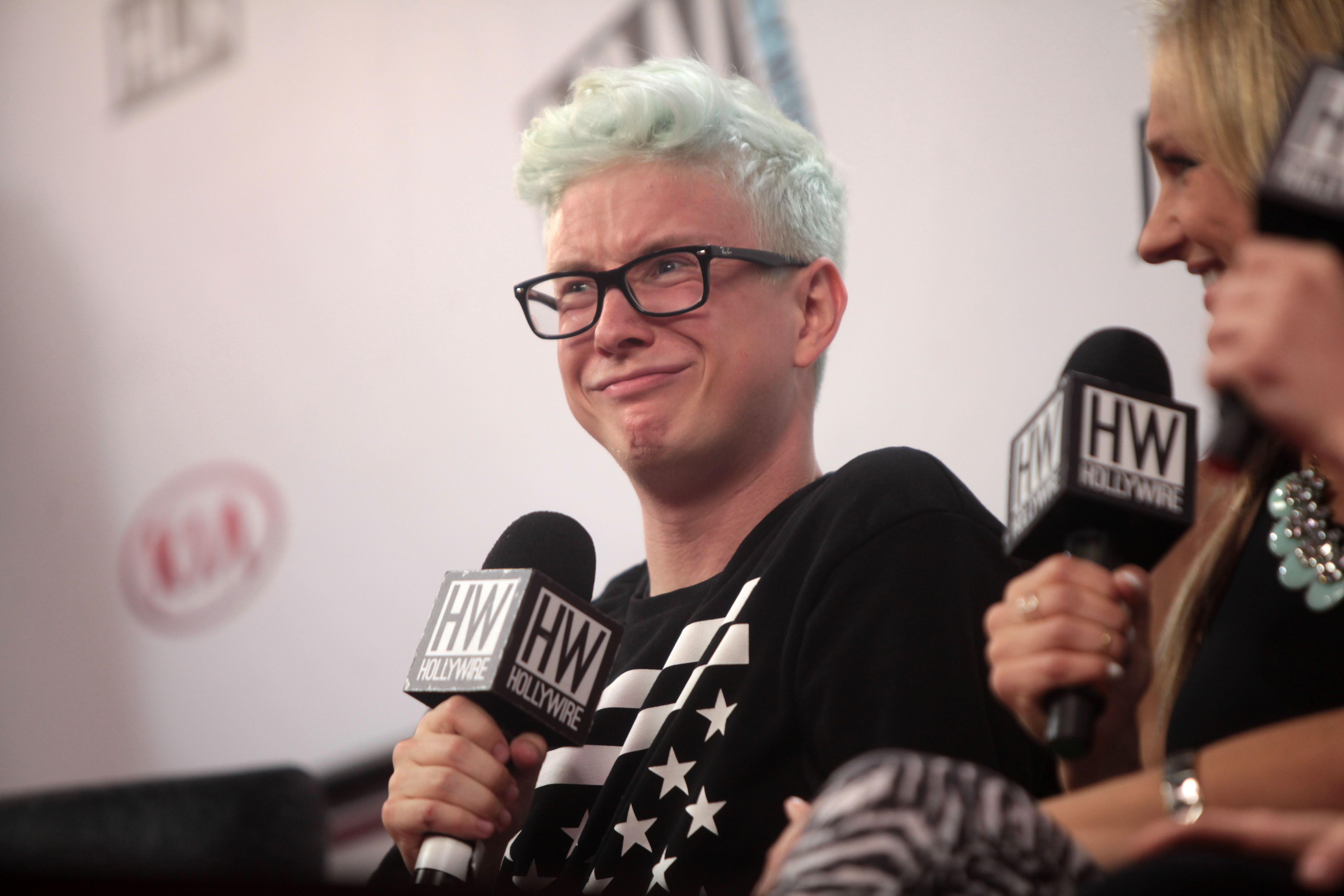The image features a man and a woman sitting and giving an interview. The man, with short white hair and black-ribbed glasses, is positioned in the center, facing slightly to the left. He is wearing a black T-shirt adorned with white stars and stripes. Holding a black microphone in his right hand, the microphone features a white square with "HW" in black letters and "Hollywire" underneath. The man appears to be cut off just below the midsection. To his right, a blonde woman is seated and looking in his direction, smiling. She is holding a similar black microphone in her right hand and is wearing white pants with black stripes. A bracelet adorns her left wrist, and she is also wearing a green and silver necklace, along with a silver ring on the second finger of her right hand. Behind them, another hand holding a microphone is visible in the background. The backdrop is a white wall or board with blurry symbols, including what appears to be a Kia logo.